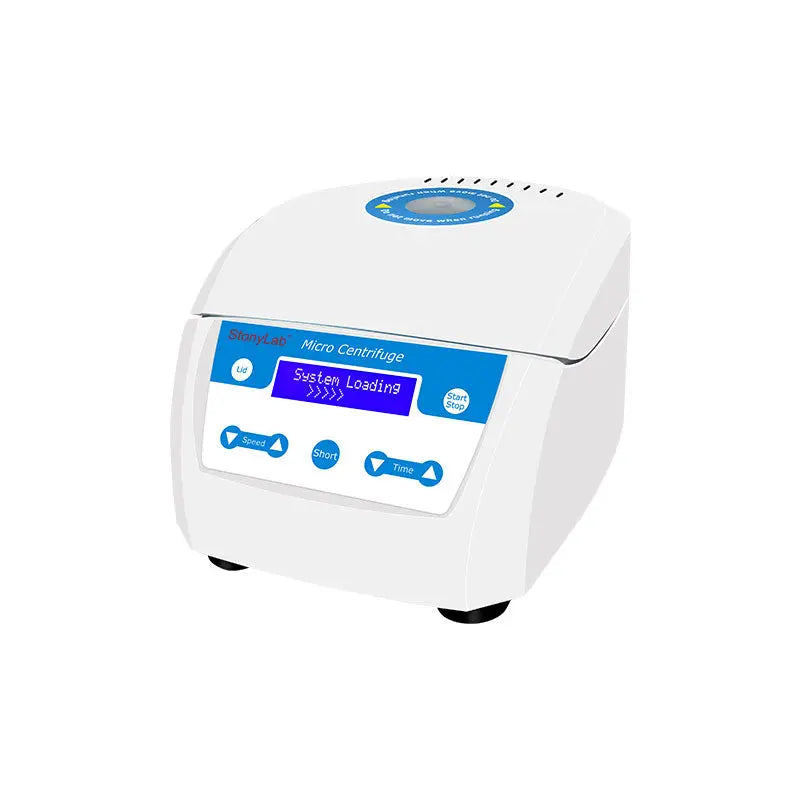This image showcases a white micro centrifuge machine, likely designed for laboratory use, placed against a solid white background, reminiscent of a product listing for online sales. The front of the machine features a prominent half-blue, half-white label where "Stony Lab" is inscribed in black lettering on the blue section, and "micro centrifuge" in white lettering on the adjacent white section. Below this label is a digital display with a blue background that reads "system loading." The device has several buttons: on the right side, a button labeled "lid," on the left side, buttons labeled "start" and "stop," all in white with blue lettering. Additionally, below these controls, there are buttons to adjust the speed and time, also featuring up and down arrows. The micro centrifuge is somewhat rounded and rectangular, evoking the shape of a small appliance like a rice cooker, and includes a circular window on the top lid. This sophisticated and compact piece of equipment, with its streamlined design and intuitive interface, is ideal for use in medical, chemistry, or biology laboratories.